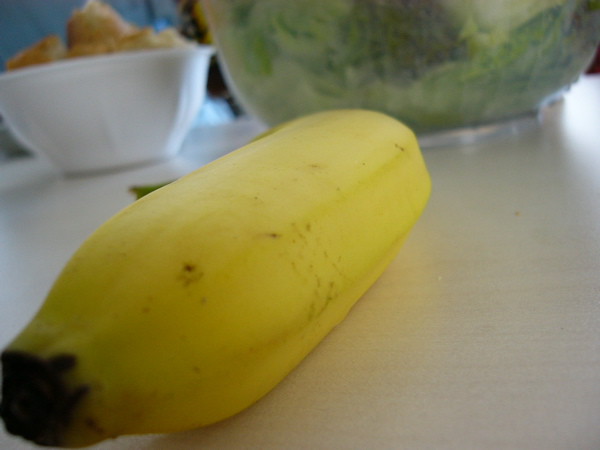A vibrant yellow banana, prominently positioned on a light-colored countertop, dominates the foreground of this image. The banana, slightly curved with hints of black and brown spots, indicates it is at the peak of ripeness. Its green stem peeks out from behind the curve, adding a fresh touch. In the background, a slightly blurred bowl filled with green lettuce and another white bowl, possibly containing cereal or another food item, are visible. The countertop contrasts sharply with a bright blue backdrop, enhancing the focus on the ripe banana and its detailed texture. The overall scene suggests a snapshot of a kitchen counter briefly capturing the fresh produce and daily breakfast setup.